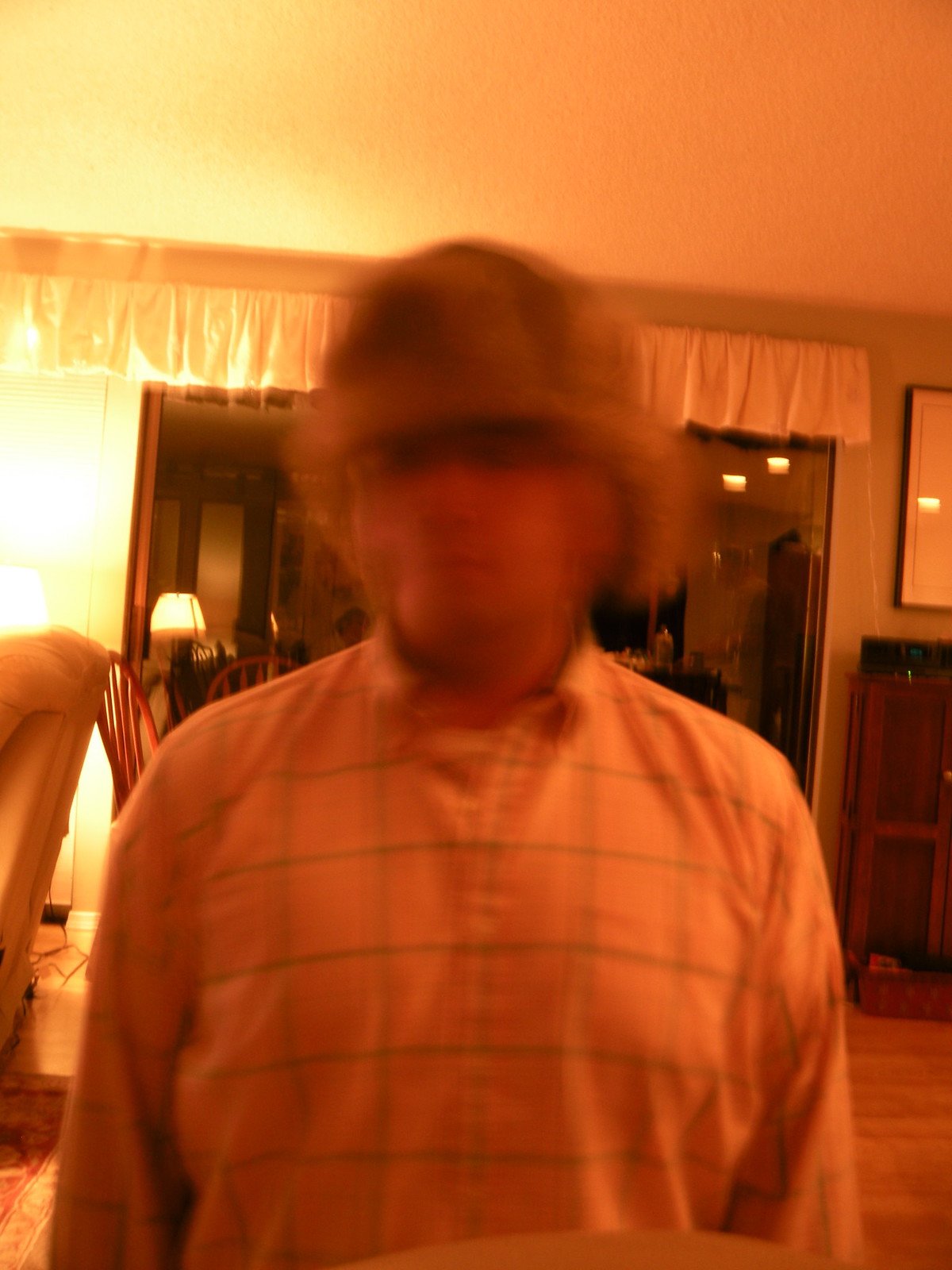In this indoor image, a man with a blurred face, wearing glasses, looks directly at the camera. His facial hair resembles a beard, and he is dressed in a button-down shirt with a grid pattern of thin vertical and horizontal lines, possibly in shades of pink and blue. The room is warmly lit, creating a welcoming ambiance. To the left of the man, a bright light stands out, while to his right, there is furniture including a cabinet with a dark top, and a framed picture without discernible details. Behind him, a large window or glass door reveals the dark night sky outside, with brown chairs and a table visible beyond. The room also features a valance over the windows and a recliner or the backside of a couch, along with brown wooden flooring, contributing to the cozy setting.